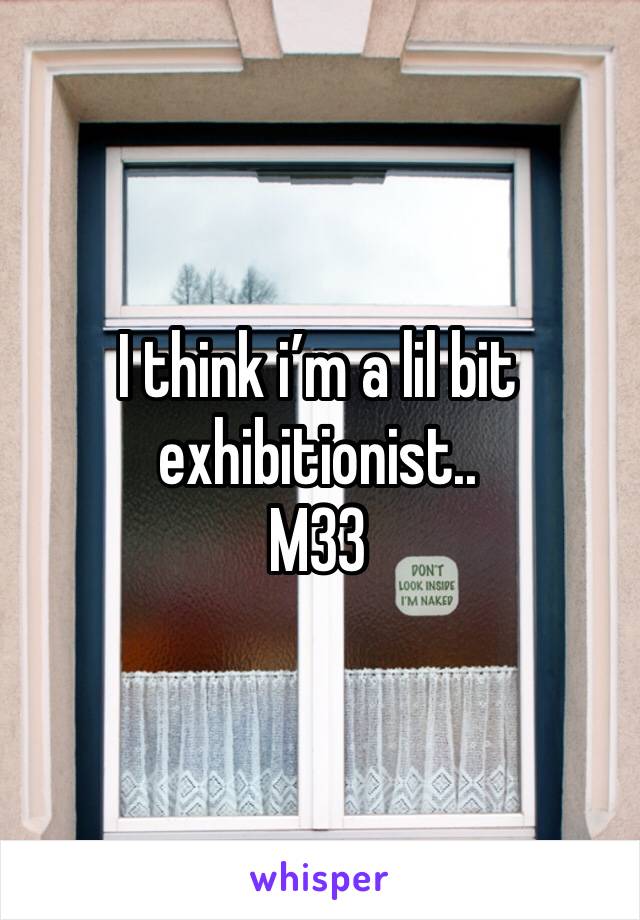The image depicts a vertically rectangular, deeply inset window encased in a light beige concrete wall that juts out, creating a recessed effect. The window features a distinct dark navy blue frame with white interior trim. It consists of two sections: an upper horizontal rectangular pane with reflective white borders revealing treetop reflections, and a lower larger vertical pane, bisected by a white divider. A set of white lace curtains with a diamond pattern decorates the bottom half of the lower window section.

Prominent white text overlays the window, stating, "I think I'm a little bit exhibitionist, M33." Additionally, a smaller sign attached to the window warns, "Don't look inside I'm naked." Completing the visual at the bottom in purple, lowercase text is the word "whisper."